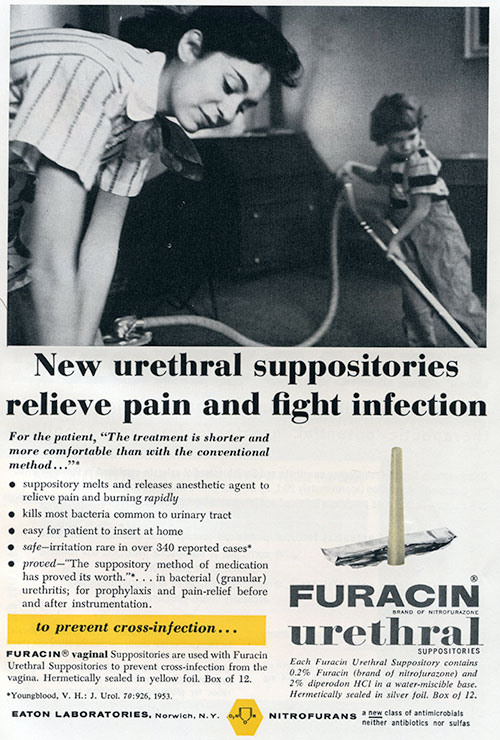This advertisement, likely from the 1960s, features a black and white photograph occupying the upper half of the page. The image shows a domestic scene where a woman, with dark hair pulled back and wearing a short-sleeved, striped Peter Pan collared shirt, is bent over, presumably cleaning. Only her upper back, arms, and head are visible as she looks down. Beside her, a young child with shaggy hair and baggy pants is holding the hose of an old-fashioned, heavy, chrome vacuum cleaner. The background reveals dark wood furniture and other indistinct items, creating a mid-20th-century ambiance.

Beneath the photo, bold text announces: "New Urethral Suppositories Relieve Pain and Fight Infection." In smaller italics, it promises, "For the patient, the treatment is shorter and more comfortable than with the conventional method." A detailed bullet-point list follows, highlighting the product's benefits:
- Suppository melts and releases an anesthetic agent to relieve pain and burning rapidly.
- Kills most bacteria common to the urinary tract.
- Easy for patients to insert at home.
- Safe: irritation is rare in over 340 reported cases (citing the Journal of Urology, 1953).
- The suppository method has proved its worth in bacterial granular urethritis for prophylaxis and pain relief before and after instrumentation.

A yellow band below the list emphasizes, "To prevent cross-infection," referring to the use of Furrison Vaginal Suppositories in conjunction with the urethral version. The lower part of the ad features an image of the urethral suppository alongside its foil wrapper. At the bottom, the manufacturer's information is presented: "Eaton Laboratories, Norwich, NY," accompanied by a yellow hexagon symbol and the term "Nitrofuranes" in bold text, identifying the active component.